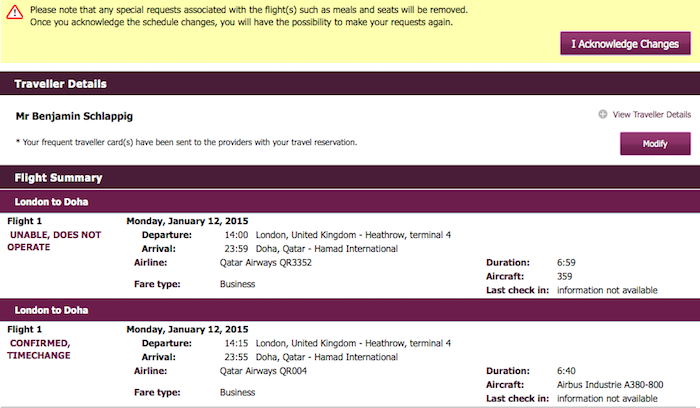The image depicts a section of a web page with several distinct elements. The background is primarily white, featuring horizontal bars in deep purple and dark brown colors that section off various parts of the page. 

At the very top, there's a yellow frame containing a message in black text: "Please note that any special requests associated with the flights such as meals and seats will be removed. Once you acknowledge the schedule changes, you will have the possibility to make your requests again." 

To the right, inside a small purple window, there is a button labeled "I acknowledge changes."

Moving down, the next section provides traveler details, displayed in white text on a gray horizontal bar. Below this, the name "Mr. Benjamin Schlapeg" is prominently written in black text.

Further down, there is a flight summary section. "Flight Summary" is written in white on a dark brown bar. The rest of the image details flight summaries, including information for a journey from London to Doha, with the flight details written in white on a deep purple bar.

The overall design is clean and functional, with distinct sections allowing easy navigation and readability.